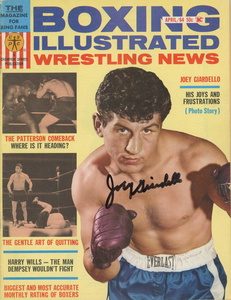This is a detailed magazine cover description for an issue of "Boxing Illustrated," with the vibrant yellow background setting the stage. Prominently displayed at the top in blue is the publication's name, "Boxing Illustrated," followed by "Wrestling News" in bold red. Along the left side, there are two vertically stacked black and white photos of men in a boxing ring. The top photo is captioned "The Patterson Comeback, Where Is It Heading?" and the bottom one, "The Gentle Art of Quitting." Beneath these photos is a headline in black, "Harry Willis, the Man Dempsey Wouldn't Fight," followed by an additional comment in red about the magazine’s reputation as "the biggest and most accurate monthly rating of boxers."

Dominating the right half of the cover is a large, full-color image of a muscular boxer in a fighting stance. He has short, curly brown hair and is wearing shiny blue Everlast shorts with a white waistband, along with red boxing gloves. This boxer, identified as Joey Giardello, has signed his name across his image in black ink, adding a personal touch. Above this photograph, in the top left corner, is a smaller note declaring the magazine as "The Magazine for King Fans." The juxtaposition of the vintage black-and-white photos against the vibrant color image creates a compelling snapshot of boxing history, capturing an era's spirit and its celebrated fighters.